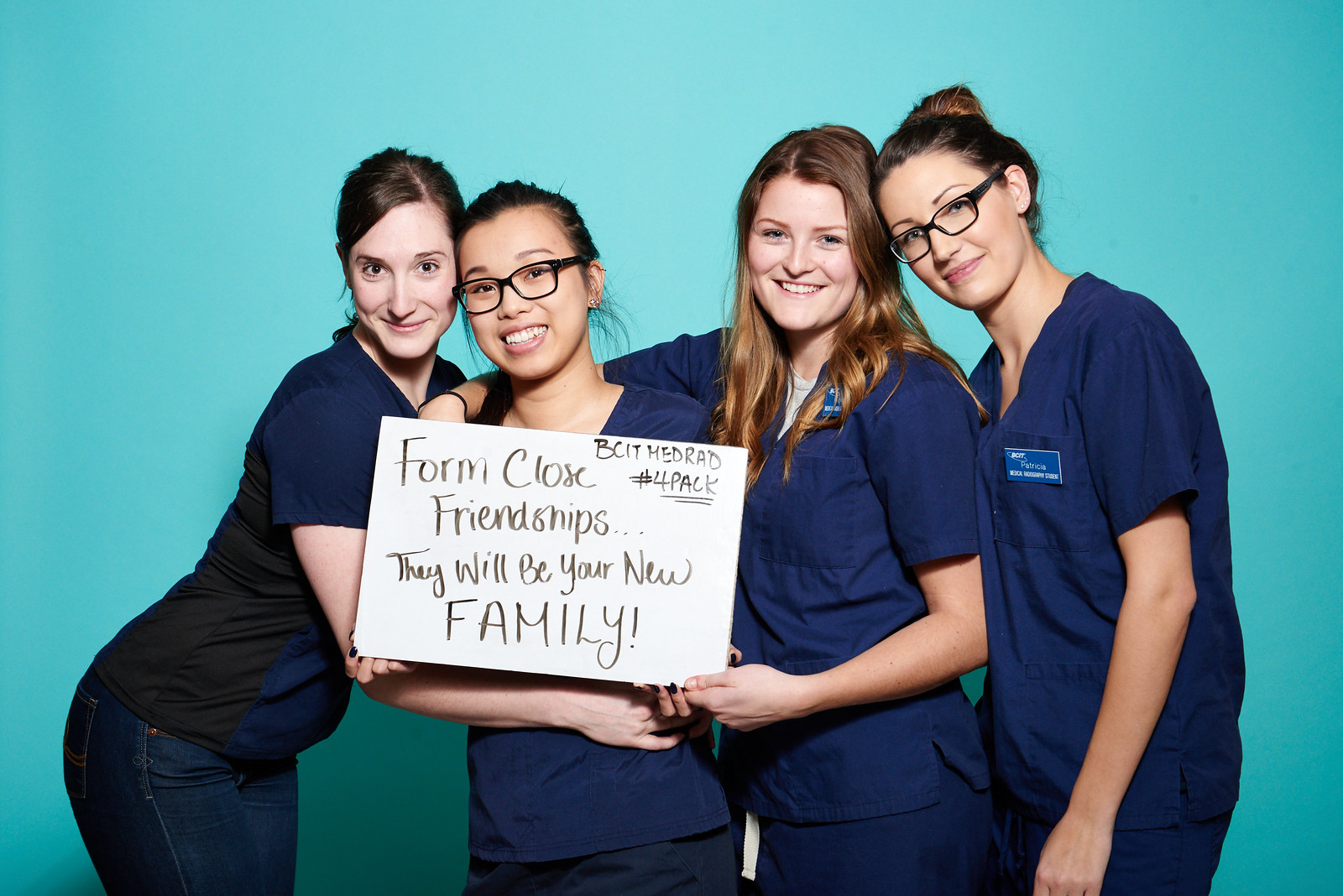In this horizontally aligned rectangular picture, four young women, who appear to be nurses or nursing aides, are standing closely together, smiling warmly at the camera. They are all dressed in navy blue scrubs, with the exception of the woman on the far left, who is wearing a navy blue top with a black back and blue jeans. The group appears united and friendly, as three of the women have their arms around each other and two of them are holding a white rectangular sign. The sign, written in marker, reads: "Form close friendships, they will be your new family." Across the top of the sign, it says: "BCIT MED RAD #4PACK," emphasizing their close-knit group identity.

The background of the image is a solid, light Easter-blue color, which contrasts crisply with their navy blue attire. Details such as blue name tags with illegible white text are visible on the left chest area of the two women on the right. The woman on the far right has her hair pulled back in a bun and is wearing glasses. The next woman to her left has long light brown hair, while the third woman has black hair pulled back and is smiling broadly with glasses on. The woman on the far left has her hair tied back and has light brown hair.

Ethnically, the woman on the far left is white, the second woman from the left is Asian, and the remaining two women are white. Their youthful energy and friendly demeanor suggest they are in their twenties.